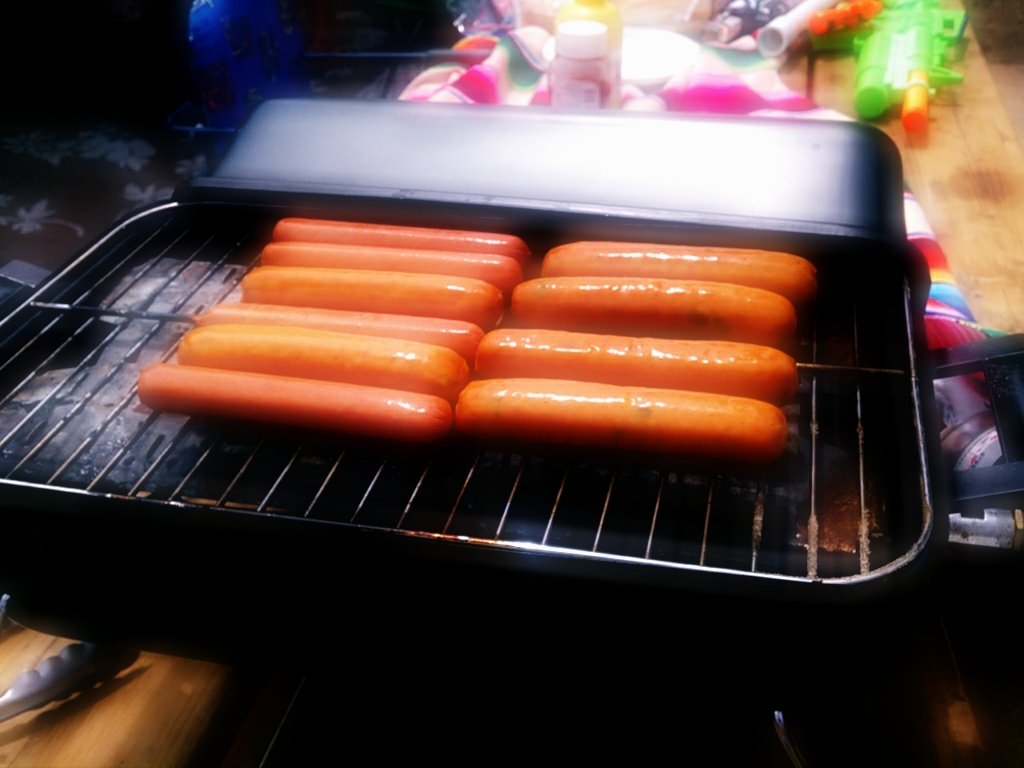This is a detailed photograph of an outdoor cookout scene centered around a small, black portable barbecue grill. The grill, slightly rusted and dirty, dominates the frame and sits on a medium-wood picnic table with a colorful tablecloth that has a bright pink and rainbow pattern. On the grill are ten hot dogs, glistening with grease and freshly placed, arranged in two rows with six on the left and four on the right. The grill’s silver grate reveals charcoal or possibly gas flames beneath it. The grill lid is propped open along the back edge. In the bottom left corner of the photo, a pair of silver tongs is visible. The background features an array of picnic essentials including a bottle of ketchup and mustard, and a green super soaker water gun with an orange spout. There is a hint of a possible Hawaiian palm tree print visible at the top left of the image, which could be part of clothing or a blanket. A blue camp chair is situated at the left edge of the table, further enhancing the casual, festive ambiance of the cookout scene.